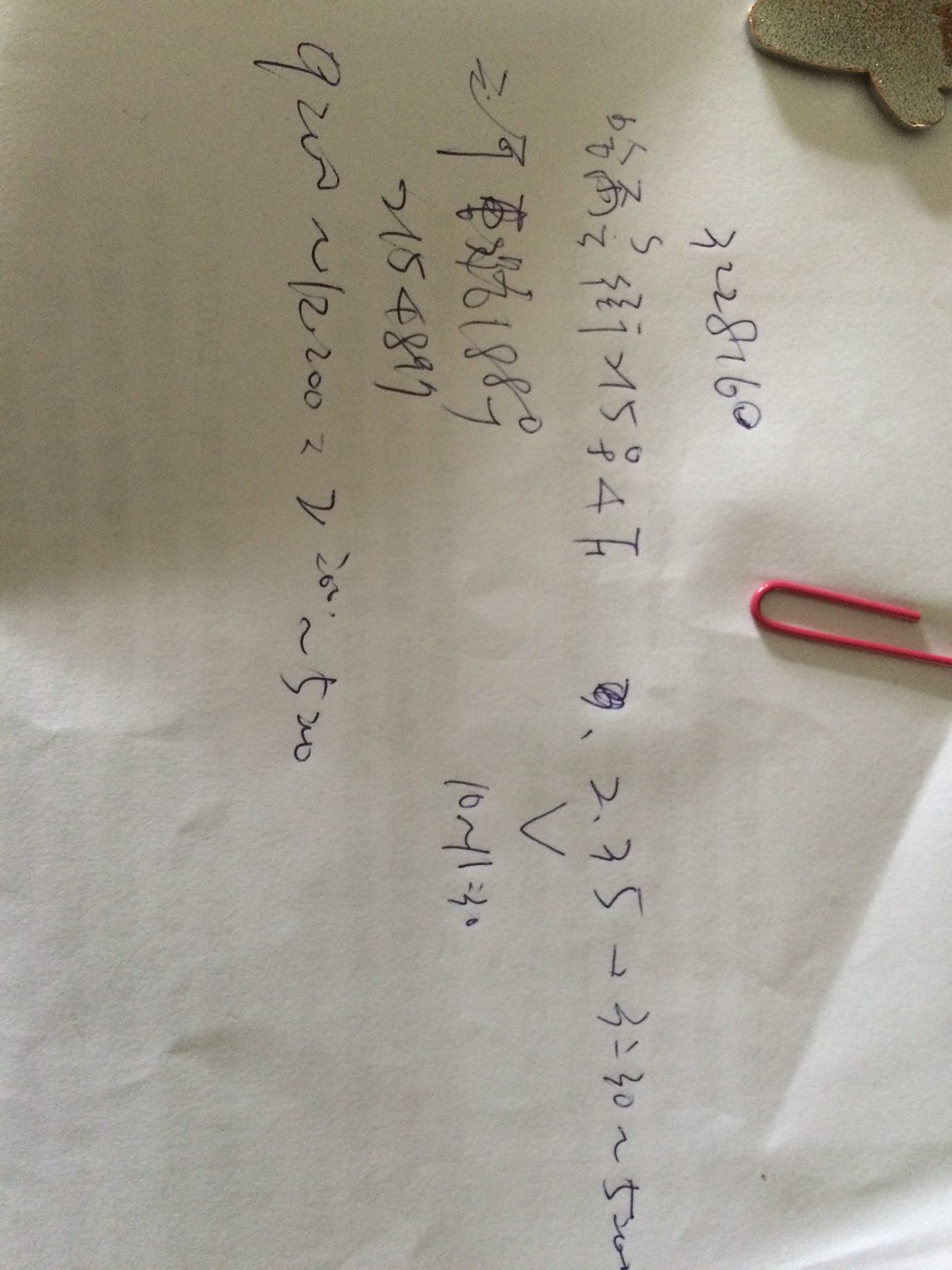The image depicts a piece of paper with cursive Korean script and the number 160, rotated 90 degrees clockwise. Positioned in the center, a hot pink paperclip partially visible (about three-quarters) creates a crease in the middle of the paper. In the top left corner, there is an indistinct clip-like object with a gold glitter color. The Korean script begins to the left of the pink paperclip, followed by the number 160. Below this, there is additional Korean text, a space, some numbers, more Korean text, and an arrow pointing down towards more Korean script. On the left side, another segment of Korean script roughly half the length of the initial text is visible, accompanied by two more lines at the bottom. The final line extends halfway across the paper, surpassing the pink paperclip. Additionally, there appears to be writing faintly visible on the opposite side of the paper.